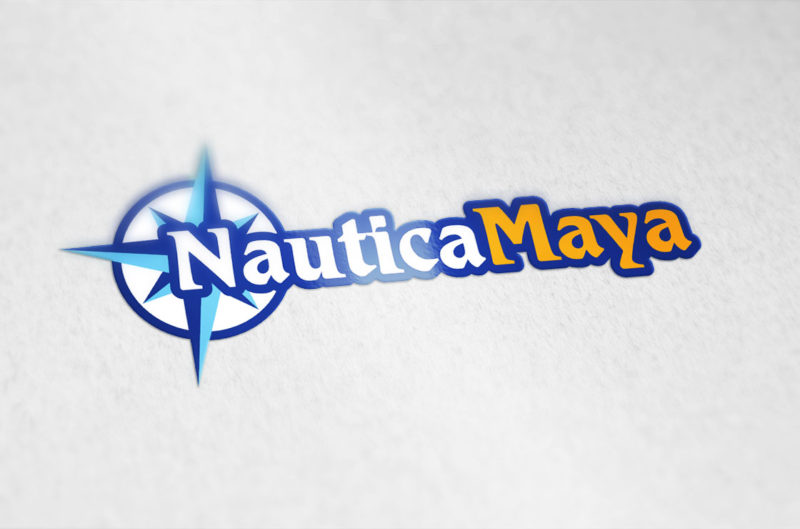The image depicts a fabric, possibly a t-shirt, with a textured grayish-white background that resembles the look of a popcorn ceiling. Central to the design is the logo "Nautica Maya." The word "Nautica" is rendered in bold white letters, outlined in dark blue, and slightly faded, suggesting wear. Following seamlessly is "Maya" in a vibrant orange hue, also outlined in blue. Positioned behind the initial letters 'N' and 'A' of "Nautica" is a compass icon. The compass consists of a filled blue circle featuring a cross and an X, wherein each cardinal direction is thicker, and colored in a gradient of light to dark blue. Notably, the top part of the compass appears blurry, in contrast to the sharply defined lower elements.